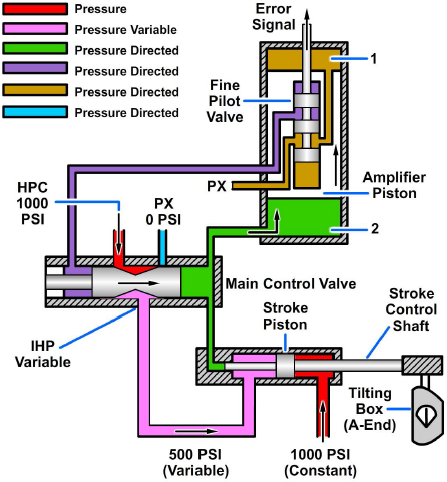The diagram is a detailed illustration of a fluid system featuring various pipes and valves, outlined with a color-coded legend to indicate different pressure states. At the top left, the legend uses colored rectangles with labels that denote specific pressure conditions: red for "pressure," pink for "pressure variable," and green, purple, brown, and blue for "pressure directed." The diagram on the right shows sections of the fluid system corresponding to these colors, illustrating the flow dynamics through the pipes. Key components labeled in the diagram include a main control valve, stroke piston, stroke control shaft, amplifier piston, a fine pilot valve, and an air signal. Arrows within the diagram depict the direction of fluid flow, and various machinery involved is also highlighted. The diagram also references units such as PSI (pounds per square inch), indicating the pressure measurement within the system.